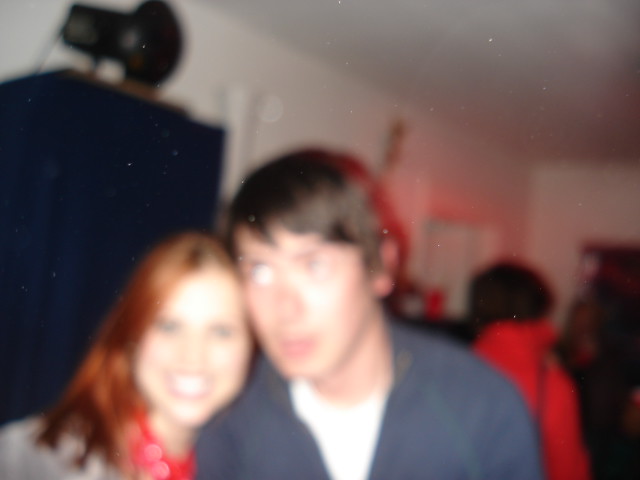This very blurry photograph depicts a man and a woman, presumably a couple, standing close together with their heads touching as if posing for the camera in a cozy setting that might be a bedroom. The man, who has short brown hair with bangs, appears to be wearing a blue jacket over a white t-shirt. His facial expression is neutral or slightly disengaged, as he looks off to the right, possibly rolling his eyes or looking up at something. His complexion appears Caucasian with a reddish hue. Next to him, the woman with shoulder-length red hair is smiling broadly, displaying her teeth and blue eyes. She is dressed in a red top with a floral print paired with a gray sweater. In the somewhat visible background, there are a few other figures, including a lady seen from the back wearing a red jacket and carrying a pocketbook, her brown Afro-styled hair noticeable. On a cabinet above the couple, there seems to be an indistinct object that resembles a mushroom dance light.